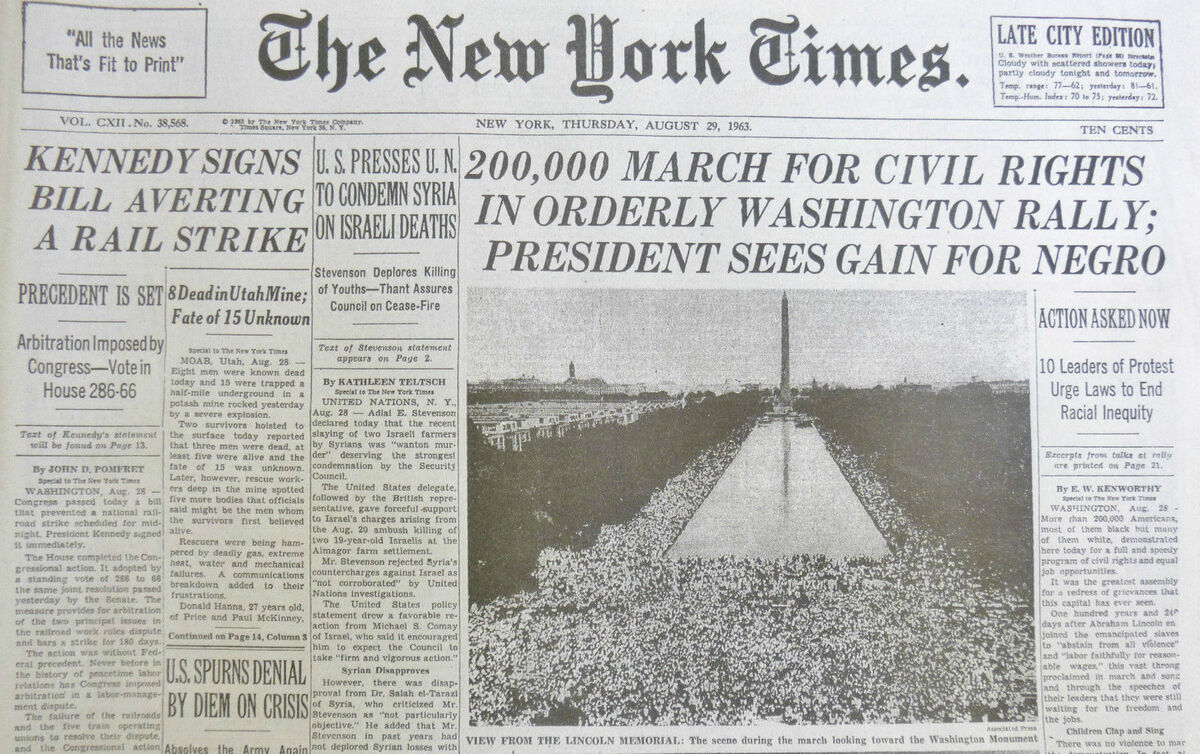This grayscale photograph vividly captures the front page of an old edition of The New York Times, dated Thursday, August 29th, 1963. The iconic New York Times masthead is prominently displayed at the top. Dominating the page is the powerful headline: "200,000 March for Civil Rights in Orderly Washington; Leaders Gain Praises from Kennedy." Beneath this major headline, a striking black-and-white image of the Lincoln Memorial spans a significant portion of the page, with an immense crowd gathered around the Washington Monument, reflecting the monumental scale and unity of the civil rights movement.

To the left, several noteworthy articles catch the eye, including "Kennedy Signs Bill Averting a Rail Strike," "U.S. Presses U.N. to Condemn Syria on Israeli Deaths," and "U.S. Spurns Denial by Diem on Crisis." On the right side of the front page, another significant headline reads, "Action Urged by 10 Leaders to Protest; Urge Laws to End Racial Inequity." This historic front page captures a momentous day in civil rights history, reflecting the political tensions and social movements of the era.